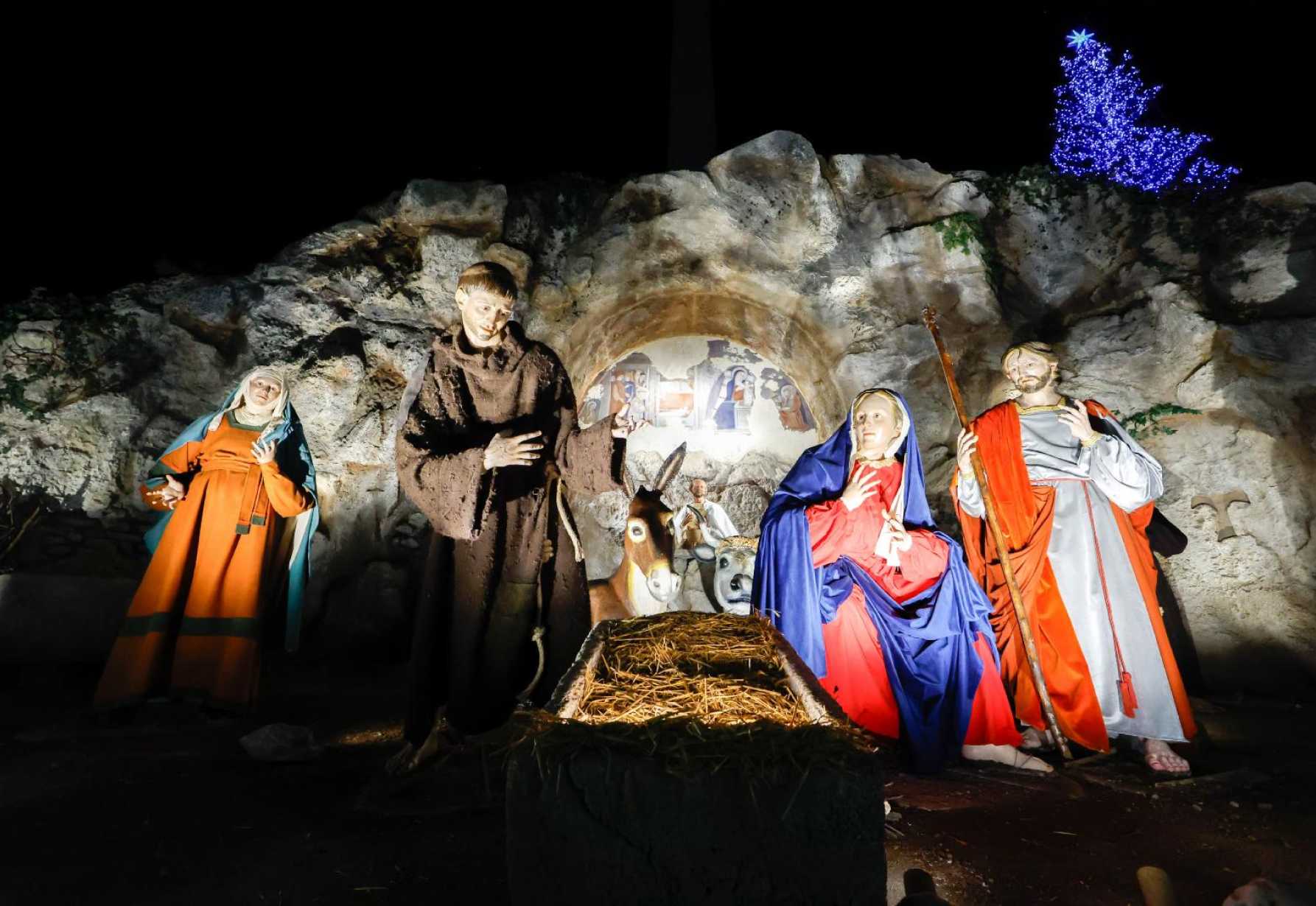The image captures a detailed nativity scene in a dimly lit environment, framed horizontally, with various elements illuminated by subtle lights. At the center of the composition is the manger, which holds hay and gives a glimpse of baby Jesus. The scene is backdropped by a large, rugged rock wall that resembles the side of a mountain, emphasizing the rustic setting.

In the foreground, slightly to the left, stands a woman in an orange dress with a blue shawl and a white head wrap; her pose is expressive, her right hand resting on her hip while the other adjusts her shawl. Beside her, a man dressed like a monk looks down into the manger, his right hand near his chest. Positioned down and to the right, a brown donkey with white markings stands beneath the neck of a gray bull, whose head is just visible behind the woman’s silhouette.

To the right of the nativity centerpiece, Mary sits in a red dress and blue cloak, her blonde hair peeking out. Her hands are raised toward her face in contemplation. Behind her, a man holding a wooden staff in his right hand, dressed in a greenish-gray robe with an orange overlay, gazes at the scene, his stance directed toward the viewer.

The background is punctuated by a small, lit-up Christmas tree in the top-right corner, adding a festive glow to the dark night sky. The entire tableau is subtly illuminated, casting gentle shadows that enhance the serene atmosphere of this Christmas manger scene.